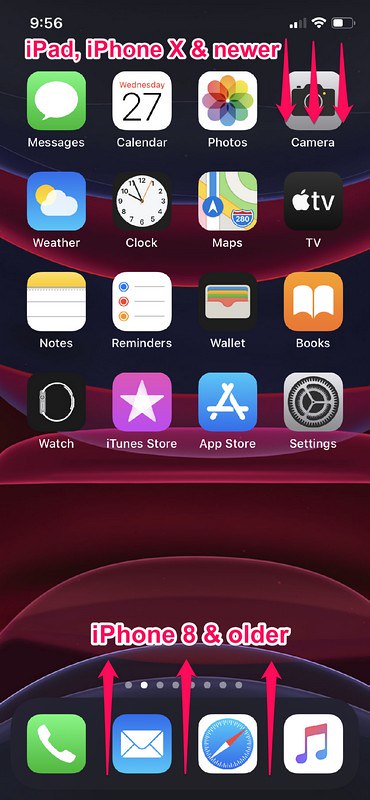A screenshot captures a mobile device's home screen, presumably from an iPhone. At the top, the text "iPad, iPhone, and X and newer" is displayed alongside three downward-facing arrows, likely indicating supported devices. Conversely, at the bottom, "iPhone 8 and older" is accompanied by upward-facing arrows. The screen showcases various app icons including App Store, Settings, Books, Wallet, Clock, Maps, Photos, Weather, Notes, Messages, Calendar, and Camera. Positioned at the bottom of the screen are core apps: Phone, Email, and Music. The background features an abstract design with overlapping circles and lines in hues of purple, burgundy, black, and fuchsia. The status bar at the top right corner shows the current time as 9:56, a battery level at approximately 50%, and a Wi-Fi connection with two out of three bars.